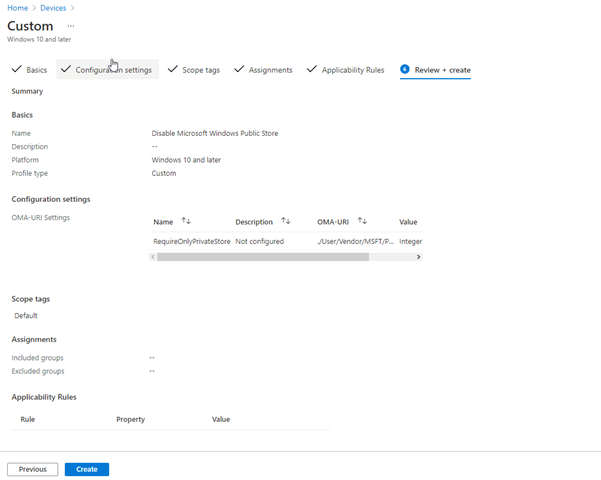The webpage has a minimalistic design with an entirely white background, giving it a somewhat monotonous appearance that suggests it may be part of the Microsoft ecosystem. 

In the upper left-hand corner, there is a breadcrumb navigation path displayed in blue font: "Home" followed by a right arrow, "Devices" followed by another right arrow, and finally, in larger, all-black, capitalized font, the word "CUSTOM." Beneath this header, in smaller gray print, it says "Windows 10 and Later."

The page features five clickable tabs, each with a black checkmark next to its title: 
1. Basics 
2. Configuration Settings
3. Scope Tags 
4. Assignments
5. Applicability Rules

Adjacent to these tabs, the option "Review + Create" is underlined in blue, indicating it's a clickable element.

Under the "Basics" tab, there is a section labeled "Summary." This section lists detailed information including:
- **Name:** Disable Microsoft Windows Public Store
- **Description:** (No description provided)
- **Platform:** Windows 10 and Later
- **Profile Type:** Custom